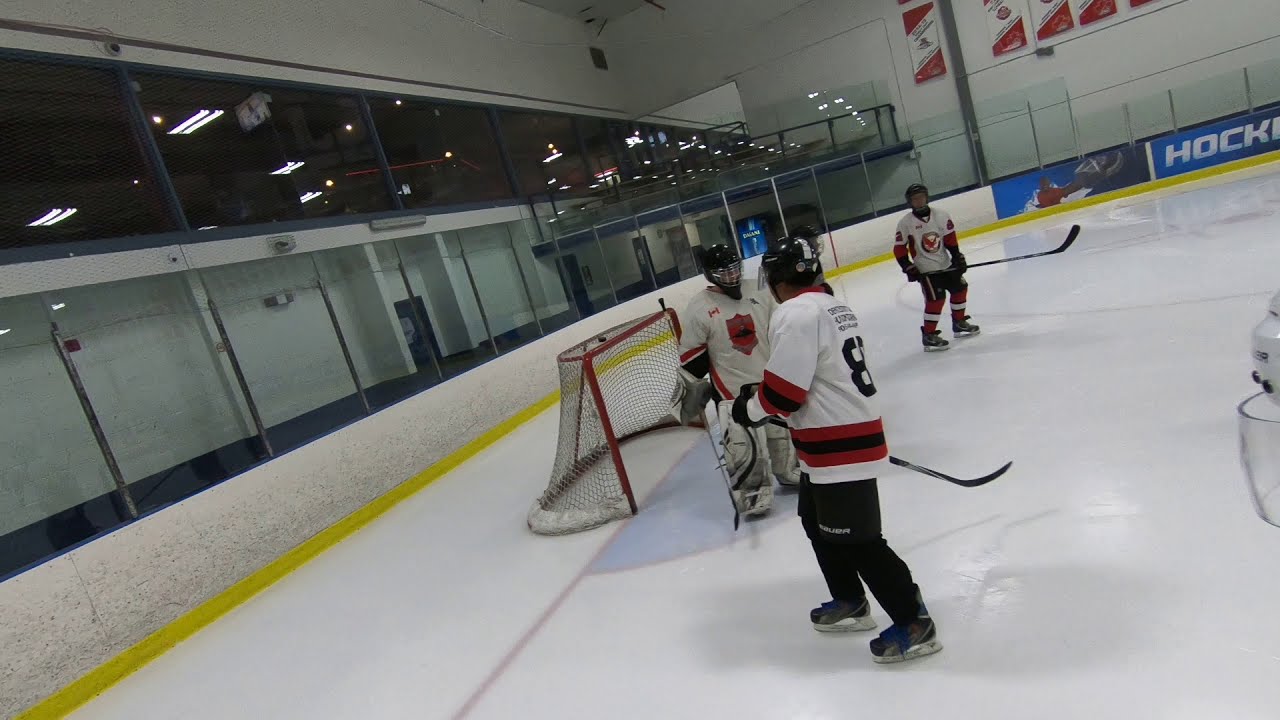The photograph captures an indoor ice hockey rink with a group of players, all donning white jerseys accented with red and black striping, black helmets, and black pants. The ice is pristine white, set against an arena devoid of spectators. Central to the image, a goaltender converses with another player, who, like his teammates, wears the same uniform. The goalie stands out with his white pants and leg padding, while another player in the background sports the uniform with black pants and red shoes. The red-framed goal with its black net is positioned to the left. The rink's structure features a yellow stripe along the bottom edge, blue and red decor on the walls, and viewing windows on the upper left side. The arena’s upper walls are predominantly white, contributing to the overall stark and clean aesthetic of the setting.